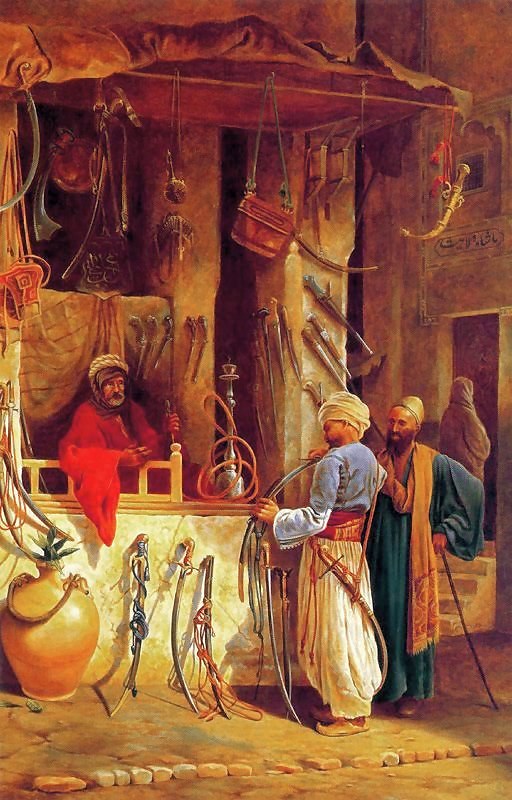The image is a detailed, cartoon-style painting set in a Middle Eastern city from the early AD centuries. It features a bustling marketplace scene with stone pathways and buildings in shades of white and brown, highlighted by the warm hues of oranges and reds. In the center, a merchant, dressed in a red robe with a tan turban and a black hood, stands between swords and a hookah displayed on his stone counter. To his right, two customers examine the wares. One shopper, adorned in a white turban, blue shirt, and gold skirt or parachute pants, holds a sword while another is strapped to his waist. Beside him, a bearded man in a tan cap and blue robe with a yellow scarf draped around his shoulders inspects the merchandise. In the background, another figure in a green and gold robe walks past the stone structures, adding depth and life to this vibrant depiction of historical trade.